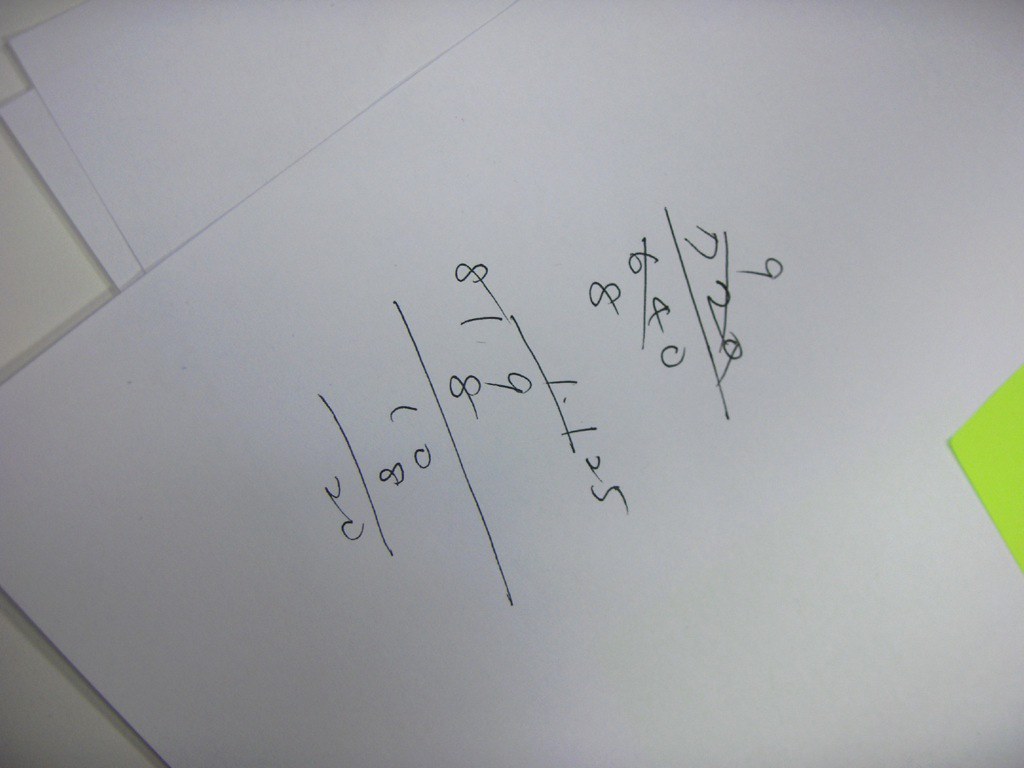This photograph captures a collection of papers, slightly askew, with handwritten notes on them. The foremost page displays a math problem, prominently featuring the equation "720 - 640 = 80". The writing is oriented from roughly 12 o'clock to 2 o'clock, indicating a slight clockwise tilt. The math appears to be a work in progress, with visible cross-outs, calculations, and corrections, including division where "9 ÷ 8" is worked out to "1.125". The writing, done in pencil or pen, is on a white sheet of paper. Beneath this sheet, several other papers are visible, arranged in various positions. On the far right-hand side of the photo, a brightly colored yellow sticky note protrudes slightly, showing just one corner. The overall scene provides a detailed glimpse into someone's problem-solving process.